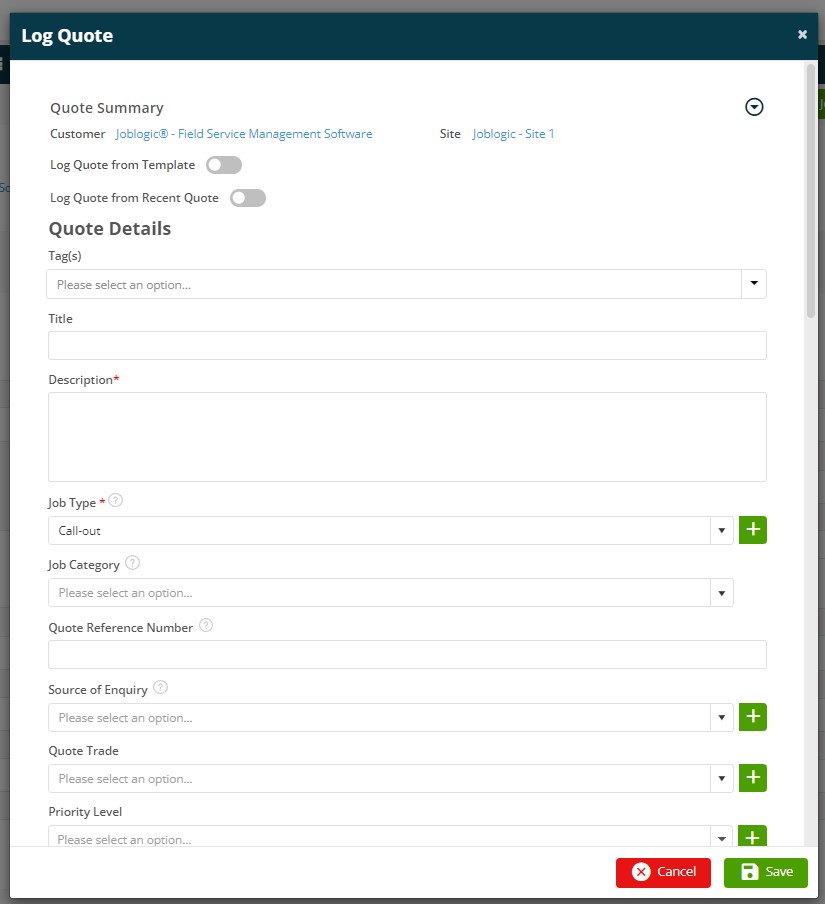This screenshot showcases a page from a Field Service Management Software titled "Log Quote." At the top, the page header reads "Quote Summary" with "Customer: JobLogic" nearby, accompanied by the registered trademark symbol (®). Below is the section labeled "Field Service Management Software" followed by "Site: JobLogic Site 1."

Further down, two options are presented: "Log Quote from Template" and "Log Quote from Recent Quote," both of which are currently disabled. The page is divided prominently into a section labeled "Quote Details" in large text.

Within the "Quote Details" section:
- There is a label "Tag(s)" with an adjacent dropdown box that says "Please Select an Option" but none are selected.
- Following this is a field labeled "Title" with a large blank text box meant for entering data.
- "Description" comes next, associated with another large blank text box.
- "Job Type" is indicated with a dropdown box currently set to "Call Out."
- "Job Category" is specified with a dropdown box that also prompts "Please Select an Option" but remains unselected.
- There is a field for "Quote Reference Number" followed by a blank input box.
- "Source of Inquiry" features a dropdown box again stating "Please Select an Option."
- "Quote Trade" is similarly presented with a dropdown box asking "Please Select an Option."
- Lastly, there is a heading for "Priority Level" followed by another selectable dropdown box showing "Please Select an Option."

At the bottom right corner of the page are two buttons: a red button with an "X" icon and the label "Cancel" on the left, and a button with a disk icon labeled "Save" on its right.